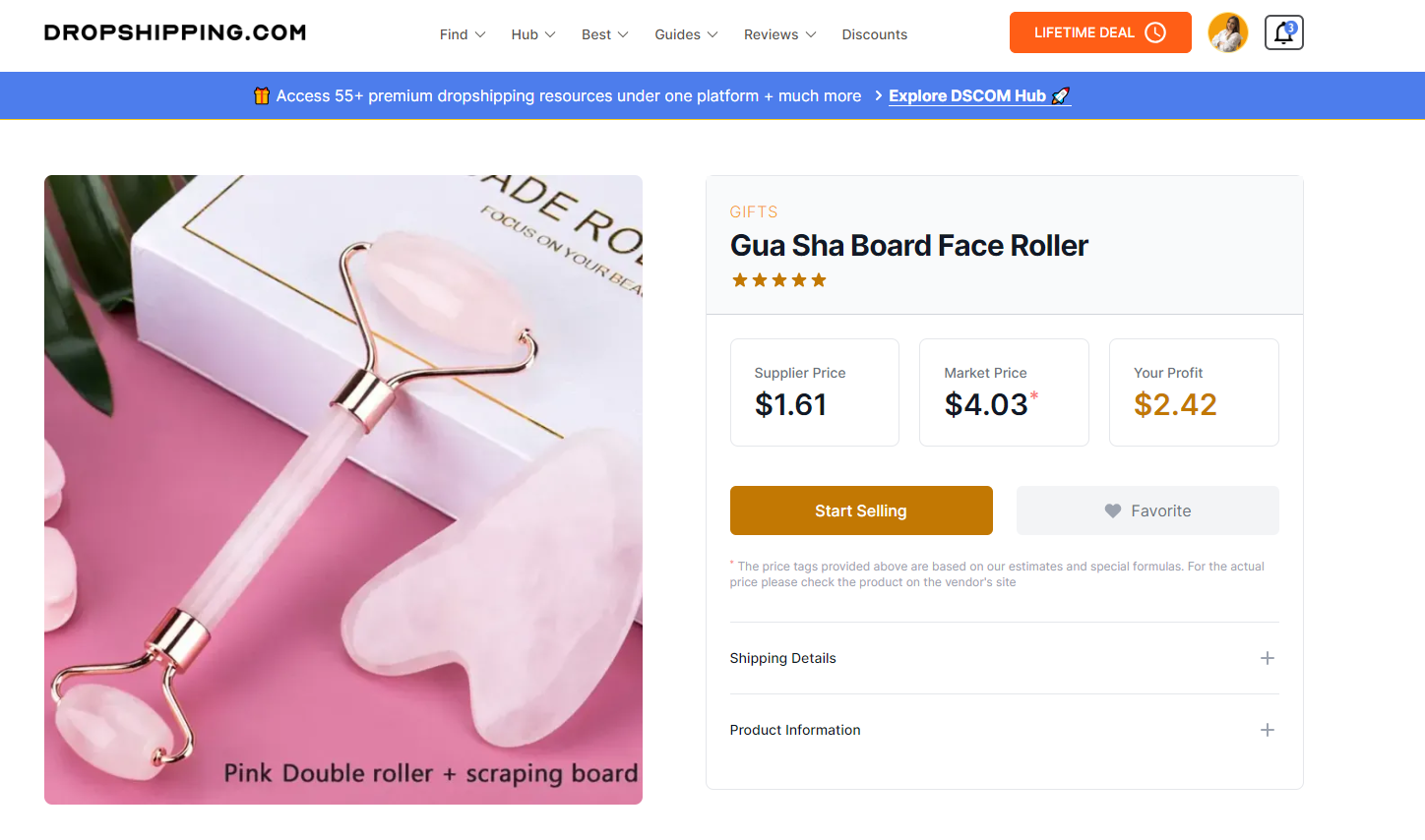This image, sourced from dropshipping.com, features the website's header and an advertisement for a product. 

At the top of the page, there is a white area that includes the website's logo "dropshipping" and a set of navigation menus labeled: Find, Hub, Best, Guides, Reviews, and Discounts. 

To the right of these menus, there's an orange box labeled "Lifetime Deal" with a clock icon. Next to it is a user profile picture of a woman with long dark hair, wearing a white shirt. Additionally, there's a notification bell displaying the number 3.

Below this, a blue rectangle stretches across the width of the page displaying a promotional banner. It features a cartoonish gift wrapped in blue and states, "Access 55+ premium dropshipping resources under one platform." Next to it, there are buttons labeled Explore, Discount Hub, accompanied by a rocket icon.

Further down, the product advertisement showcases a "Pink Double Roller and Scraping Board," described as a face roller made of pink crystal, also known as a Gua Sha board. It is priced to offer a profit of $2.42. Additional information includes shipping details and product specifications.